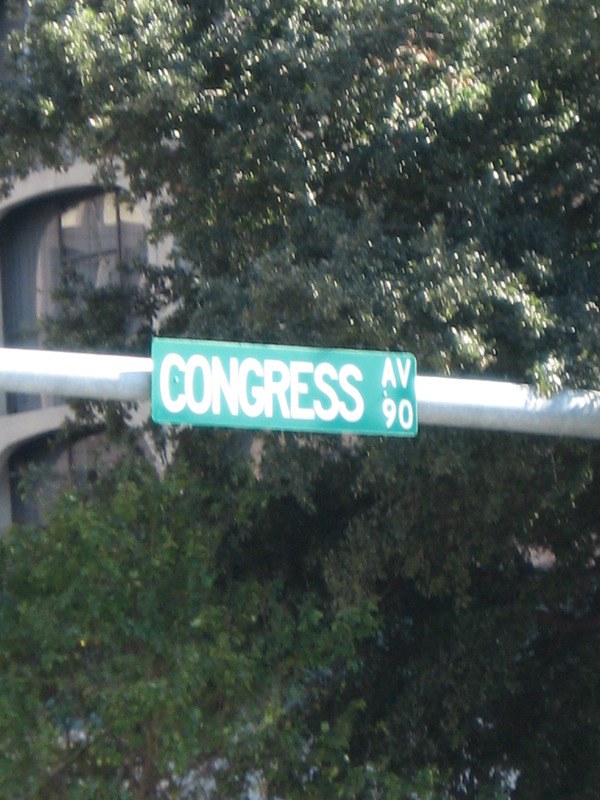This vertically-oriented image captures a street sign mounted on a probable aluminum arm that extends over a roadway, likely part of a traffic signal structure. Positioned centrally in the frame, the rectangular street sign is horizontally aligned. In the background, lush greenery from numerous trees dominates the scene, imparting a natural backdrop. The upper left corner reveals a glimpse of a residential building, adding a touch of suburban architecture to the composition. The street sign itself features the text "Congress Avenue" in prominent white letters on a classic green background, with the number "90" displayed just below the abbreviation "AV."